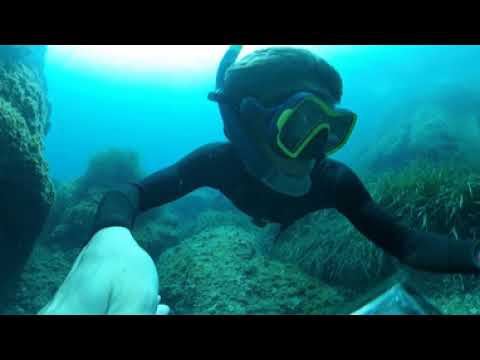In the image, a diver, likely male, is captured underwater, facing to the right but glancing to his left. He is wearing yellow and black swim goggles and a snorkel mask, with the snorkel tube visible along the right side of his face. The diver is clad in a black wetsuit or swimsuit and has his arms extended forward, creating an impression that he's reaching for something or perhaps holding a camera for a selfie. The underwater scene is vibrant with large rocks covered in algae, coral, and green sea plants, or possibly sea moss. The water is bright and clear, illuminated by sunlight shimmering from above, suggesting it's daytime with the water appearing cool and blue.